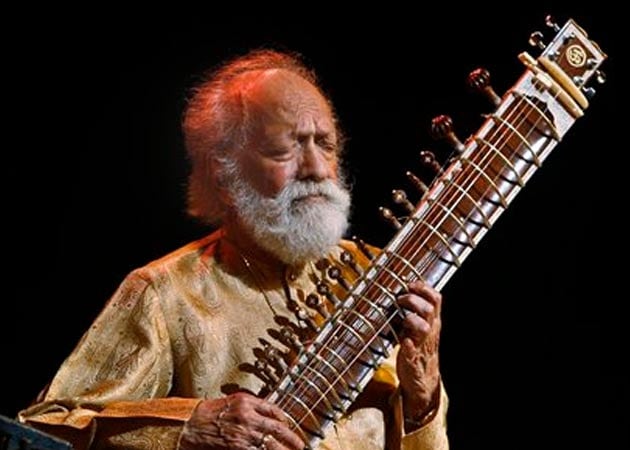This striking photographic image captures an older, white man with a balding head and a beard and mustache of whitish-gray color, deeply engrossed in playing a sitar. Set against a stark black background, the image highlights the serene and focused expression of the man, whose eyes are closed as if lost in the music. A red light casts a striking glow on his bald head, emphasizing the intensity of the moment. His face is shown in a left to right profile, looking downward. The man is wearing a gold long-sleeve shirt with hints of yellow and a ring on his right hand. The sitar, a traditional Indian string instrument characterized by its long neck and array of tuning pegs—twenty, in this case—is white and brown and features an emblem resembling an Asian character on top of the neck. The musician's left hand holds the strings while his right hand plucks them, indicating his adeptness and deep connection to the instrument. There is a palpable sense of dedication and immersion as he plays, underscored by the vivid lighting and profound simplicity of the black backdrop.